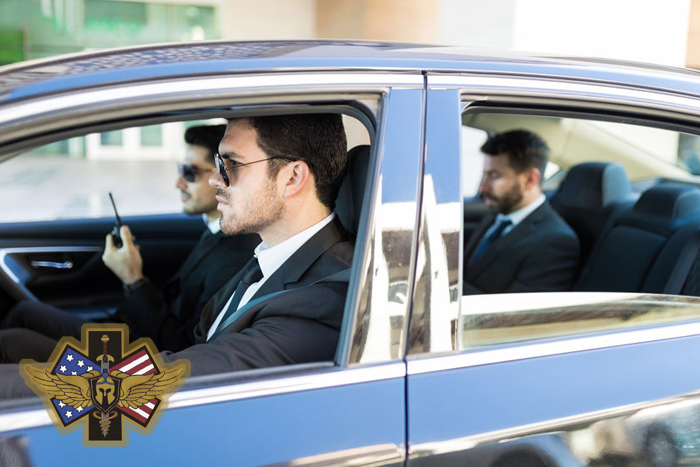The image depicts three individuals inside a car who resemble secret service or law enforcement officers. All three are donning black suits, white shirts, and black ties, with two of them wearing dark sunglasses, contributing to their serious and professional appearance. The individual in the driver's seat is focused on the road, while the person in the passenger seat is holding a walkie-talkie, hinting at their communication duties. The person in the backseat, the only one without sunglasses, appears to be looking down, possibly at a device or document. On the lower left side of the image, an emblem is visible featuring a crossed pair of American flags, a sword, and golden wings, suggesting a coat of arms or an official insignia. Additionally, the reflection of a nearby building can be seen on the car's window, adding context to their environment.